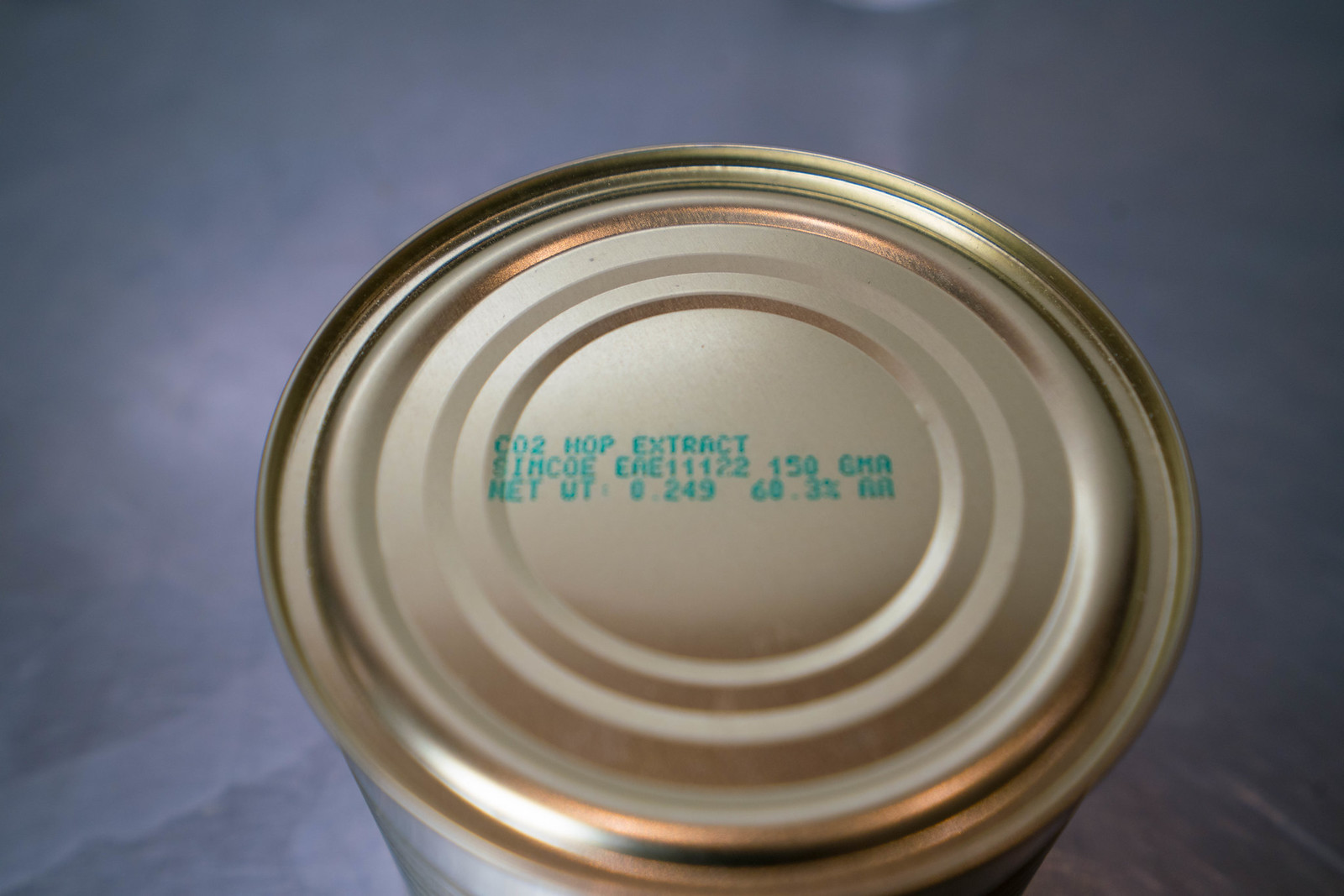The image is a close-up of the bottom of a metallic can, likely made of aluminum, with a brass-toned finish that appears slightly matte from the angle shown. The can bottom is distinctly circular with grooved concentric rings, contributing to its shiny appearance. It looks like a typical 15-ounce can, perhaps for soup or beans. The can rests against a light blue table adorned with white lines, providing a contrasting background. Green text on the bottom reads "CO2 hop extract" and "Synco 15A GMA," along with other code numbers and phrases such as "net weight 0249, 60.3 AA." The detailed codes are somewhat blurry but still legible against the can's surface.